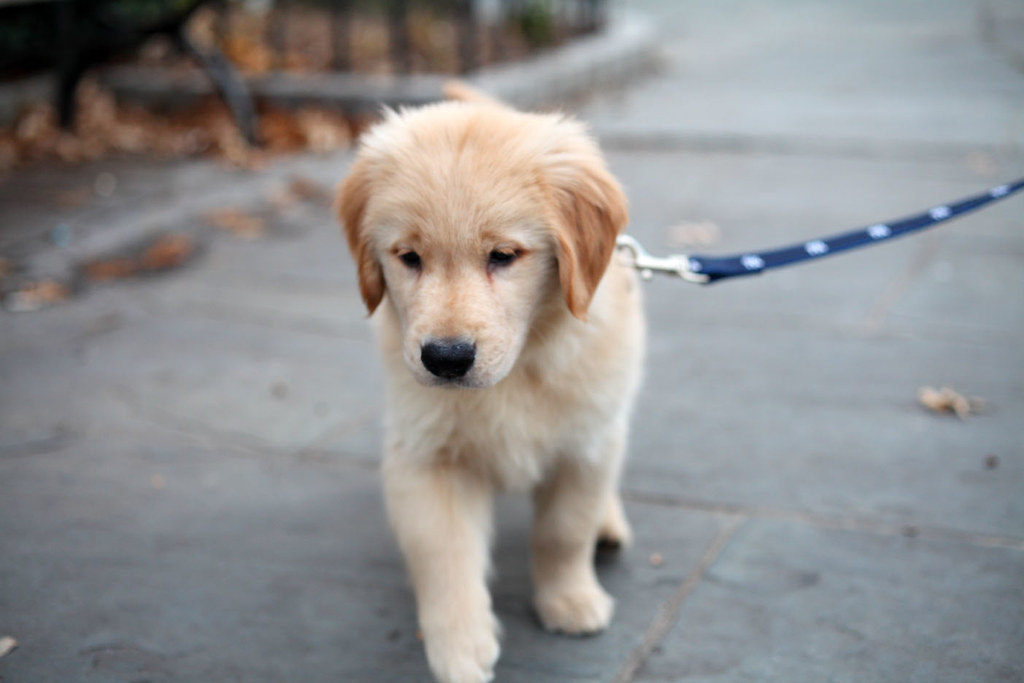A close-up photo capturing a light brown puppy walking on a sidewalk outdoors. The puppy, with darker brown dangling ears, appears to be walking towards the camera, its cute face in sharp focus while the background remains blurry. The puppy's leash, colored blue and white with a visible silver clamp, extends out to the right side of the frame. One of the puppy's paws is raised mid-step, giving a sense of motion. In the distant background, the sidewalk stretches away, flanked by a hazy fence, and scattered leaves are visible along the pathway, adding an autumnal touch to the scene.